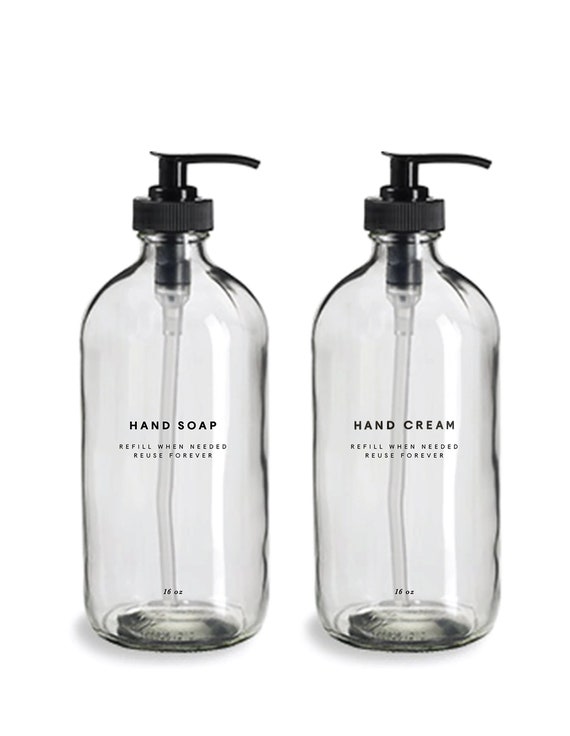This image showcases two clear 16-ounce bottles labeled "hand soap" on the left and "hand cream" on the right. Both bottles feature a simplistic and sophisticated design, emphasizing minimalism with their clean, transparent appearance and frilly text. Each bottle is topped with a black plastic pump lid and includes a clear straw reaching down to the bottom, indicating the efficient dispensing mechanism. The labels on both bottles read "refill when needed, reuse forever," highlighting their environmentally sustainable design. Although described as possibly being plastic, the subtle uneven surface of the bottles suggests they might be high-end, handmade glass. The lighting in the image is professionally set, with reflections indicating light coming from the right side, enhancing the overall polished look of the product photo.